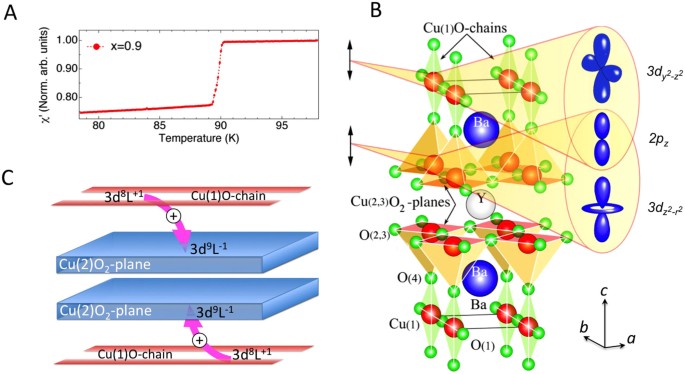This image is a detailed scientific diagram divided into three sections, labeled A, B, and C. 

**Section A**, positioned in the top left corner, features a line graph. The graph includes the labels "Norm Arb Units" on the Y-axis and "Temperature, K" on the X-axis, with temperature values ranging from 0.80 up to 1.0. The graph also has two red lines, one that runs horizontally, then jumps, and another that continues horizontally again. The letter 'A' is prominently displayed next to this graph.

**Section B** dominates the right half of the image and consists of various chemical structures and their makeup. This section includes green, orange, and red circles organized inside cone-shaped drawings, some of which are labeled, such as "Cu1" and "Cu2302 planes." There are also references to "Cu1O chains" and "molecules of green and red." The intricate details highlight different chemical compounds and their structures, represented by an assortment of colored balls and connecting chains.

**Section C**, located on the bottom left, contains four distinct colored layers with the top and bottom layers being red and the two middle layers blue. These layers are arranged with various labels attached, including chemical names, numbers, and a pink arrow pointing from the middle layer to an adjacent part. This part also includes tiles at the bottom, each labeled with different identifiers, providing additional context to the depicted structures.

Overall, the diagram presents a comprehensive view of chemical elements and their distribution, with a focus on copper (Cu) and oxygen (O2) components, showcasing both their graphical and structural details in a complex and colorful array.